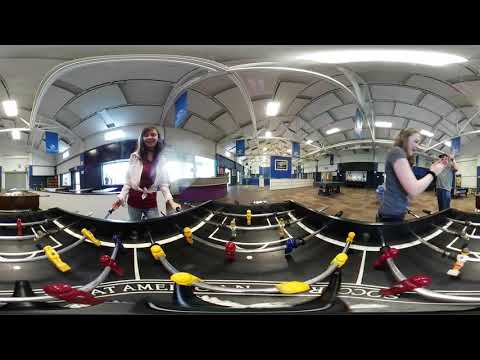In this image taken indoors at a recreational facility or sports center, two young women are engaged in an intense foosball game. The camera appears to be positioned at the center of the black foosball table, which features yellow and red figures and has white lettering, including the letters A-T-A-M-E-O-C-S. 

On the left, a girl with dark hair, wearing a red shirt underneath a white sweater, and blue jeans is focused on the game. To the right, another girl with light brown hair clad in a gray t-shirt and blue jeans is clapping her hands, possibly celebrating a recent victory. 

The background reveals a vibrant setting with various table games, including a pool table, and a counter on the left side. Overhead, the tile ceilings are adorned with bright white lights. A man in a gray shirt and blue jeans can also be seen standing in the background, contributing to the lively atmosphere of the game room or recreational area.